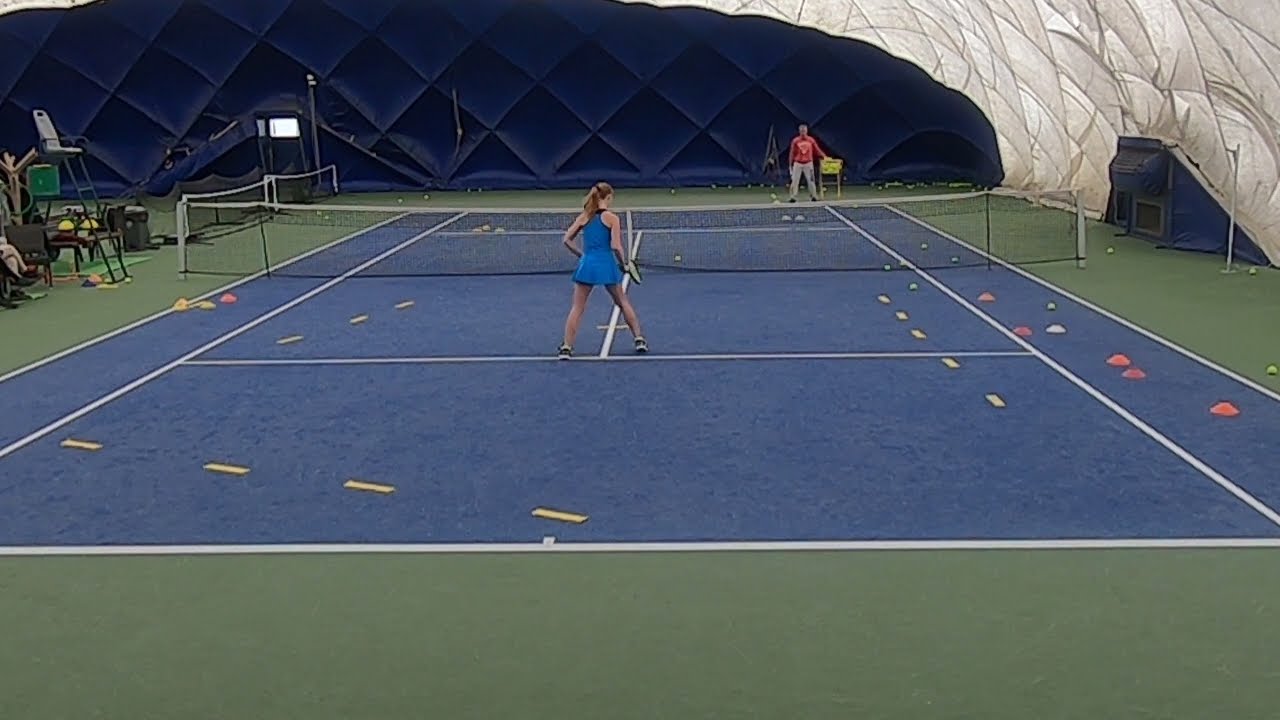The photograph captures an indoor tennis court, primarily blue with white and yellow lines, encircled by green flooring. The court features a net with a black mesh and white border. Overhead, the facility boasts a distinctive white, inflatable, grid-patterned roof, giving it a balloon-like appearance, with some sections tinged blue and white walls that let in light. 

At the forefront stands a Caucasian woman with long blonde hair tied in a ponytail, wearing a light blue tennis dress with a skirt and black-and-white tennis shoes. She is holding a neon green tennis racket with a black border. Opposite her, near the back of the court, is a man in a red shirt and gray pants, possibly her coach, standing by a yellow basket likely containing tennis balls. To the left, only partly visible are the feet of another individual, cut off from the frame, and a high chair can also be seen. The background also features a tiny window and ventilation system on the right side. This setting suggests a practice session rather than an actual game.